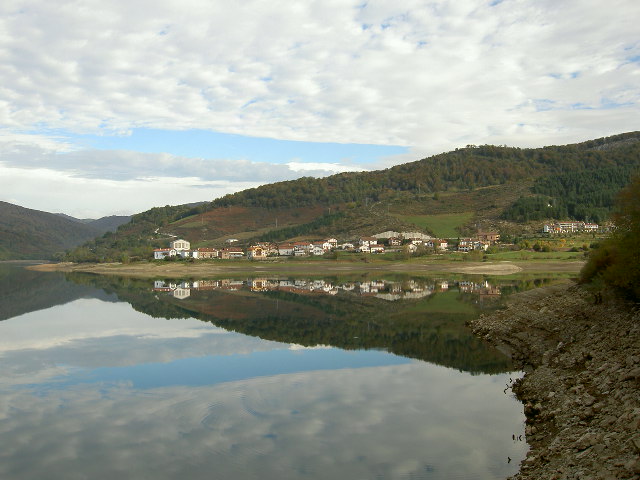This photographic image captures an idyllic outdoor scene during the day, featuring a serene lake with still water that perfectly reflects the blue sky dotted with white clouds, and the surrounding green mountains. The foreground showcases the glassy lake, while in the midground there is a collection of 15 to 20 predominantly white buildings with red, brown, and orange gabled roofs. These buildings, which make up a small community or village, stretch across the middle of the photo against a backdrop of tree-covered mountains. Of particular note, on the left side of the village is a large one-story building with expansive floor-to-ceiling windows, and on the right side stands a multi-story white building with porches. The right-hand side of the lake's bank rises to meet the foliage-covered hillside, revealing a mix of dirt and greenery. There are no people or text visible in this vibrant and tranquil landscape, making the natural and architectural elements the central focus.